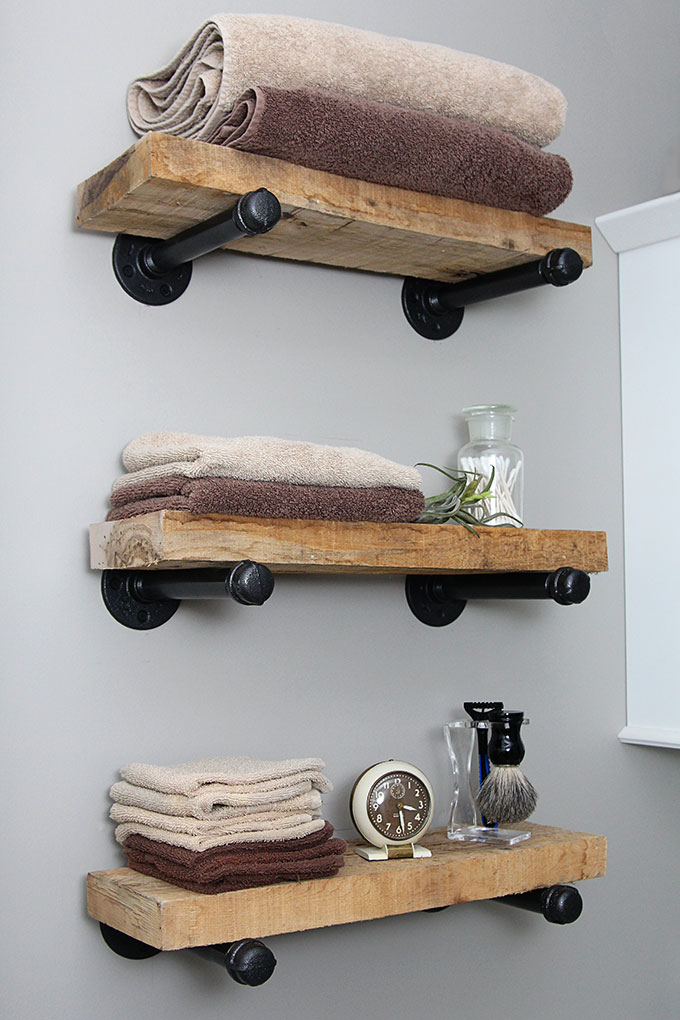This image depicts a set of three industrial-style shelves mounted on the light gray wall of a bathroom. The shelves are constructed from heavy, untreated, rough-sawn oak planks supported by black, stovepipe-painted pipe brackets with flanges and caps. Starting from the top shelf, we see neatly folded bath towels in beige and dark brown. The middle shelf holds hand towels in matching beige and dark brown hues, beside a glass jar filled with Q-tips and a small succulent plant. The bottom shelf features six washcloths—four beige and two red—a white analog clock, and a holder made of acrylic containing a brush and a razor. To the right of the shelves, there is a white cabinet mounted on the wall. The entire setup showcases an industrial-chic aesthetic in a functional bathroom space.